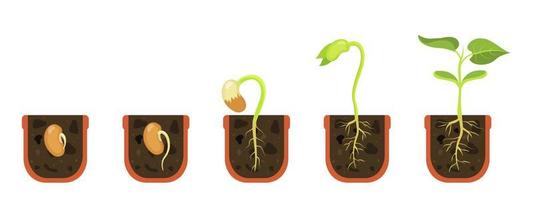This is a detailed color illustration showcasing the stages of seed germination and early plant growth, presented through five cutaway sections of small pots. Each section reveals a different phase in the life cycle of the plant, from seed to sprout.

In the first section, a brown, bean-like seed is embedded in black soil, showing the initial germination part emerging on the right side. The second section depicts the seed with the beginning of a white root extending downward into the soil. The sprout inside the seed is getting ready to emerge.

In the third section, the seed has partially emerged above the soil, with most of its brown sheathing stripped away. The root system is developing tendrils, and a stem curves upward in a shape reminiscent of the right side of a classic heart.

The fourth section shows a more elongated stem, darkening in green color, and the beginning of leaf formation at the top. The seed pod is no longer visible, while the roots have grown more extensive with multiple tendrils.

Finally, the fifth section illustrates a fully sprouted plant with a well-developed root system. The stem is strong and supports two lower leaves and two larger upper leaves, both dark green and narrow, appearing heart-shaped. This final stage shows a robust small plant with solid green leaves, indicating successful germination and growth.